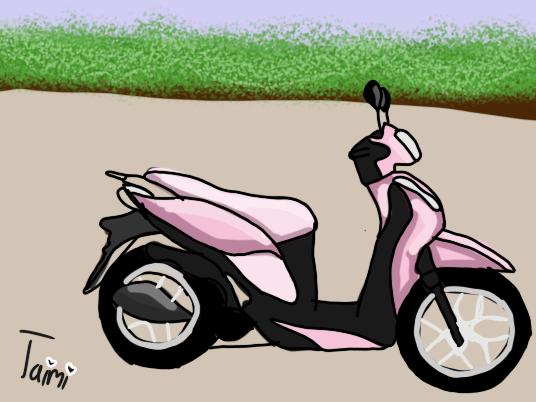The image depicts a somewhat choppy, side-view drawing of a motorcycle, or perhaps a moped, prominently painted in shades of pink and black, with white wheel spokes. This motorbike rests on a sandy beige surface with a backdrop that transitions into a dusty rose color. Beyond this, there is a bright green, grassy median that resembles either abstract leaves or grass, and at the very top of the image, a hint of a lavender sky can be seen. The scene includes some blue in the distance, possibly signifying the ocean. The artist's signature, "T-A-I-M-I," is located in the lower left-hand corner, with each "I" dotted by a heart.